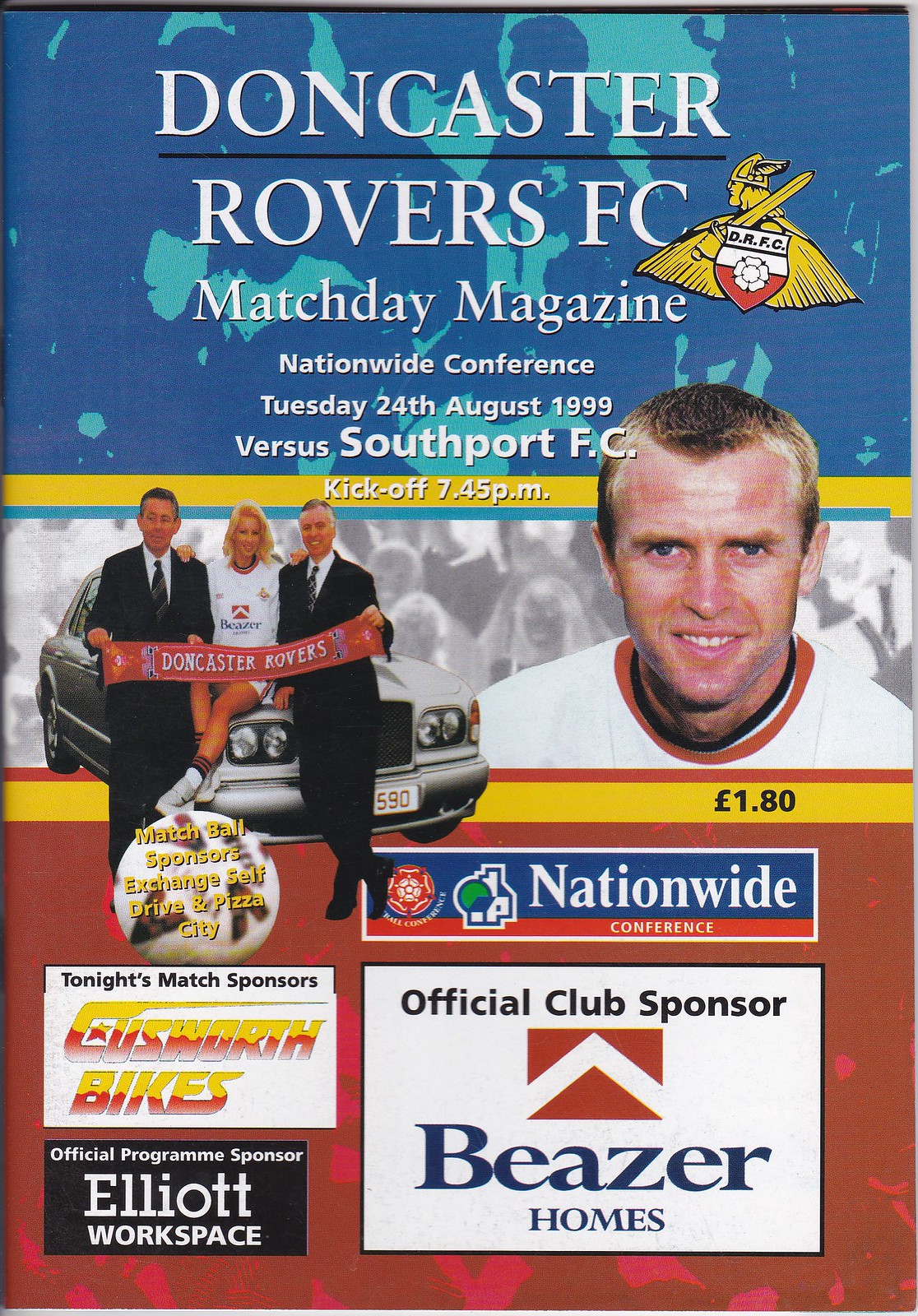The image is a detailed match day magazine cover for Doncaster Rovers FC, from a game played on Tuesday, August 24, 1999, against Southport FC, with kickoff at 7:45 pm. The cover prominently displays text announcing the Nationwide Conference, along with various sponsorships including Beezer Holmes, Nationwide, and Elliott Workspace. The magazine's background features a rich combination of blue at the top, gold accents for the club logo, and a red section below. On the left side of the cover, three individuals—two men and one woman—are seen seated on a car holding a banner that reads "Doncaster Rovers." To the right, there is a smiling Doncaster Rovers player, although his name is not mentioned. The style of the magazine is typical for a football club's match day pamphlet, encapsulating the spirit and excitement of a Doncaster Rovers FC match.